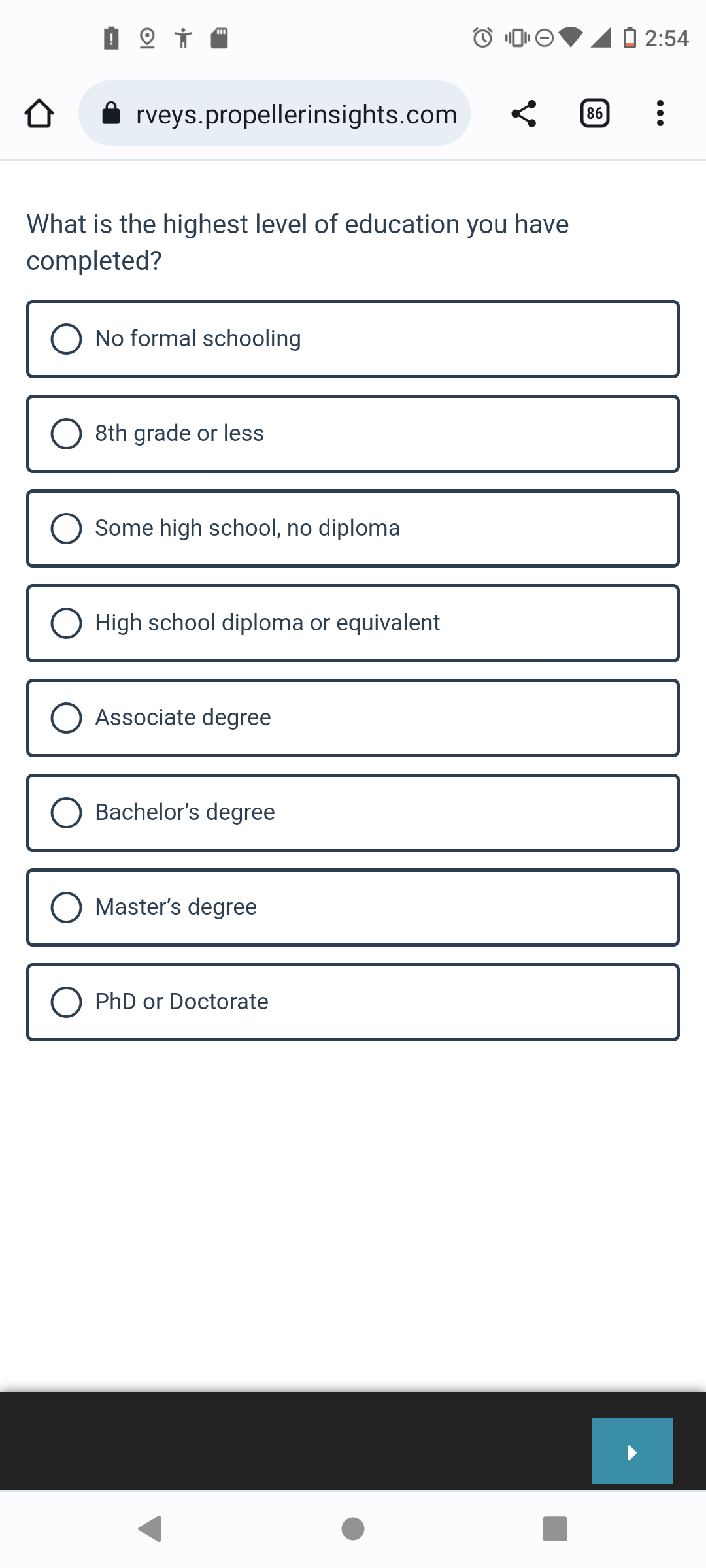This detailed caption describes an organized and precise view of a screenshot from a mobile phone. The background of the image is white, giving it a clean appearance. At the very top is the status bar displaying various icons including: a battery icon, a location sharing icon, a fitness icon, an SD card icon, an alarm clock icon, a mobile signal icon, and a Wi-Fi signal icon. The battery icon is shown again, and the time displayed is 2:54.

Below the status bar, there is a browser interface. The URL is partially visible in a gray oval and appears to be "surveys.propellerinsights.com." To the left of the URL bar is a home button, and to the right is a share button. There is also a square with the number 86, indicating the number of open tabs in the browser.

The main content of the screenshot reveals an open survey with a white background. The survey question displayed at the top is, "What is the highest level of education you’ve completed?" Following this question, there are eight selectable options presented as black-outlined rectangles. These options, listed from top to bottom, are: "No formal schooling," "Eighth grade or less," "Some high school, no diploma," "High school diploma or equivalent," "Associate degree," "Bachelor's degree," "Master’s degree," and finally, "PhD or doctorate."